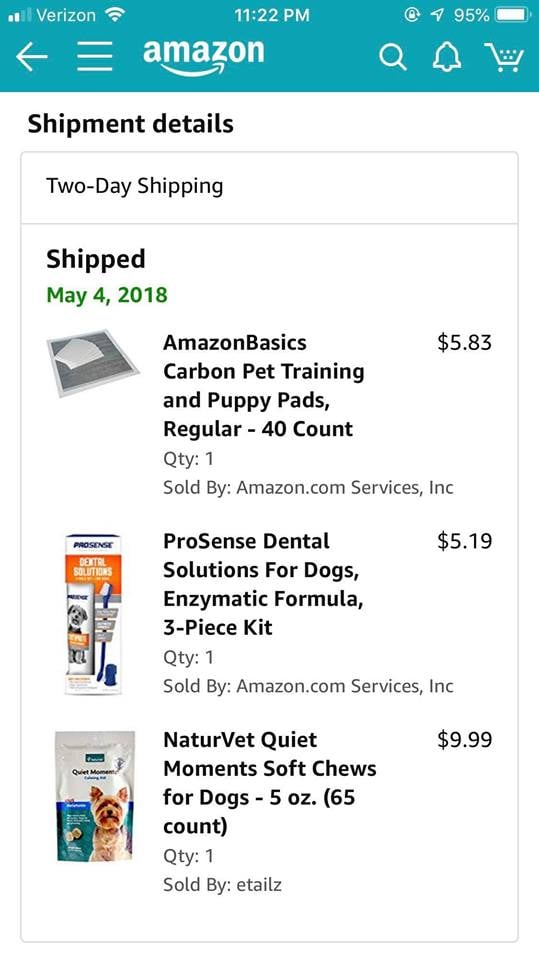This is a detailed description of a screenshot taken from someone's phone while browsing Amazon. The top inch and a half of the screen features a light bluish, almost teal blue color, transitioning to white below it. In the top left corner, two out of the four internet bars are illuminated, next to the Verizon logo in white. The Wi-Fi indicator shows a full signal, and centered on the screen is the time, 11:22 p.m. On the right side, the battery icon indicates a 95% charge, with a lock icon and an arrow next to it.

Beneath this, on the left side, there's a back arrow and three horizontal white bars stacked vertically, approximately an inch wide. Centered below is the Amazon logo in white with a small check mark below it. To the right of the logo, there are icons for search, notifications (a bell), and the shopping cart.

Just below, in the white portion of the screen, bold black text reads "Shipping details." A large black-bordered rectangle dominates the section from here to nearly the bottom of the screen. Inside the rectangle, the top left corner features "Two-day shipping" in bold black text. Below this, a line separates the text from "Shipped," also in bold black, followed by the date "May 4, 2018" in green.

The main content inside the rectangle shows a variety of purchased items. The first item listed is an image of a Puppy Pad on the left. To the right, the item is described as "Amazon Basics Carbon Pet Training and Puppy Pads, Regular - 40 count" in black text spread across four lines. Below this description, details such as the quantity, seller, and price ($5.83) are given.

The next item is a dental toothbrush for dogs, with its type, quantity, seller, and price listed similarly. The third item is a package of dog chew treats, with bold black text identifying the product. Again, the quantity, seller, and price details are provided on the right side.